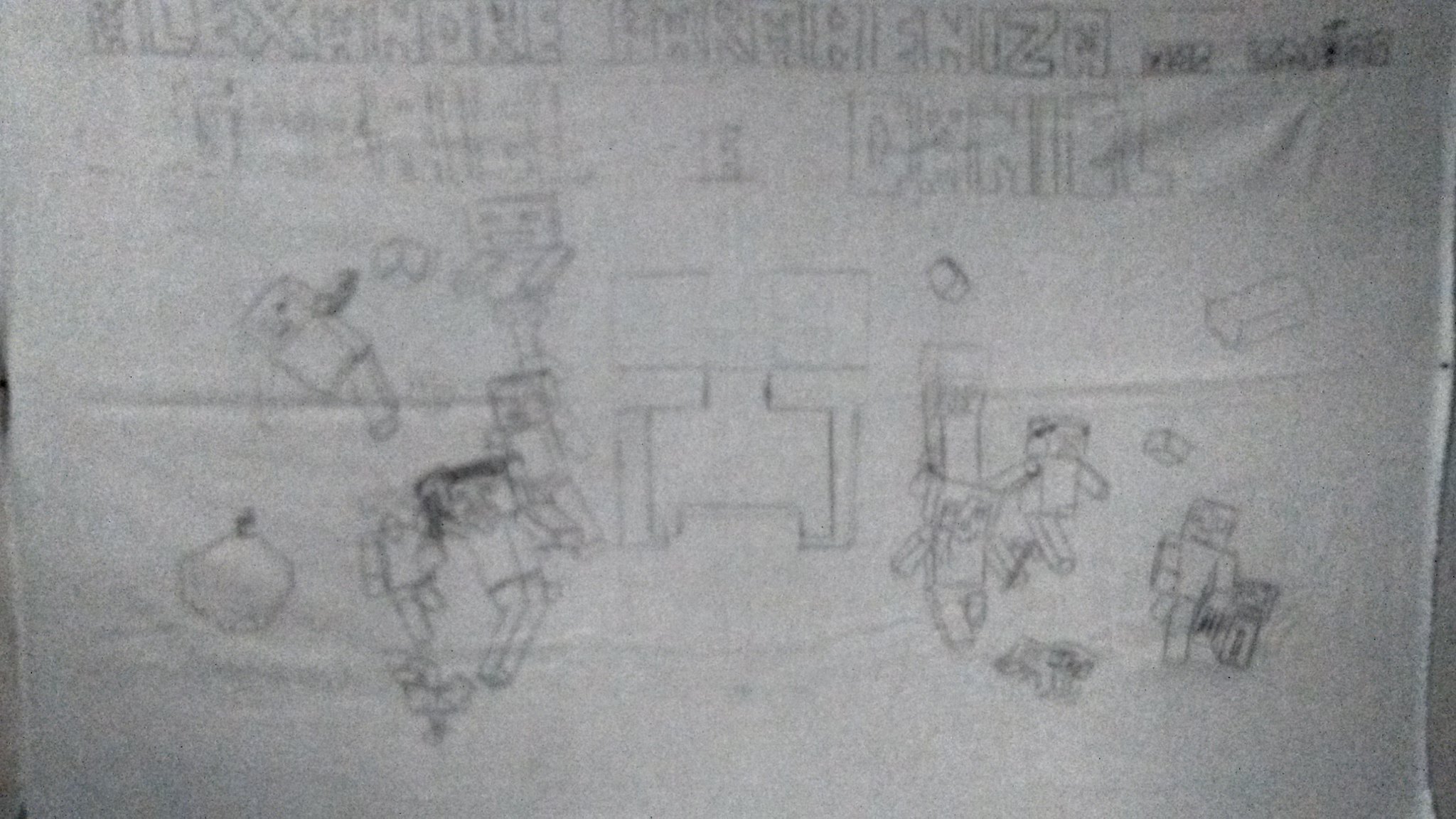This is a detailed pencil drawing done on a piece of white paper or possibly fabric. At the top of the drawing, there are two rows of block letters, though some of these letters are partially obscured or incomplete. Below the text, the artist has drawn numerous objects resembling robots. These robots feature square bodies, square heads, and rectangular limbs. The robots are depicted in various positions: some appear to be walking, while others seem to be falling. On the right and left sides of the drawing, the robots are more densely populated. In the center of the image is a structure composed of several squares stacked on top of a rectangular base, giving it a unique and prominent presence. Off to the lower left corner, there is a distinct hexagonal object, which adds an interesting geometric element to the composition. The overall artwork showcases a complex and imaginative assembly of shapes and forms.